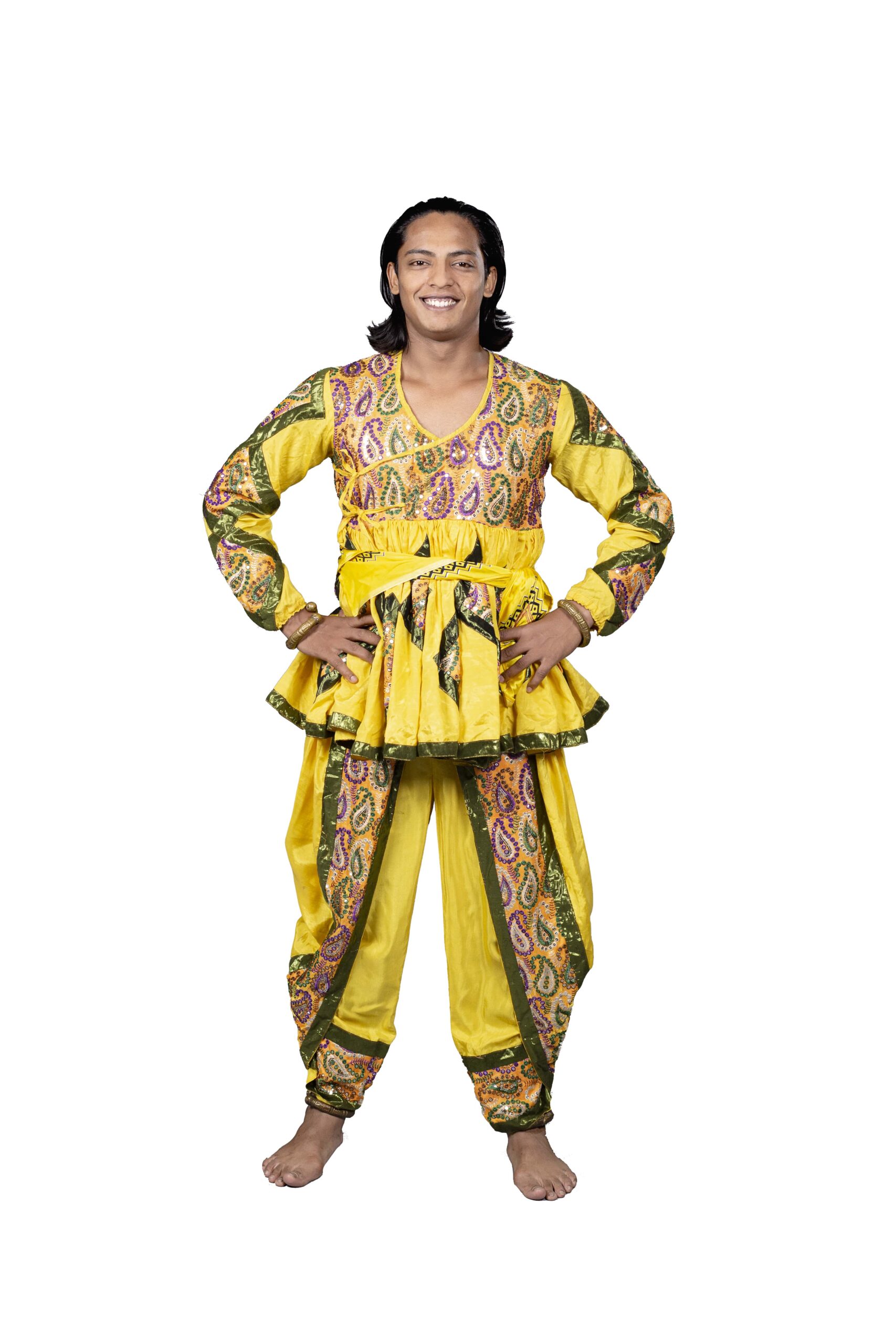A photograph features a smiling man, possibly Indonesian, standing barefoot against a completely white background. He is dressed in traditional cultural attire characterized by a predominantly bright yellow color with intricate designs. The ensemble includes a long-sleeved top adorned with a low, curved V-neck, and embellished with green bands, vibrant purple and green paisley patterns, and sequins, particularly prominent on the upper chest area. The top has a distinctive ruffled fringe at the waist, mimicking a short skirt, and is outlined in dark green. His billowy, genie-style pants feature the same yellow fabric with green and paisley design stripes running down each leg and around the gathered ankles. He has shoulder-length, dark hair combed back, revealing his brown skin. The man stands confidently with his hands on his hips, accented by a gold bangle on his right wrist, and gazes straight ahead with a broad smile.